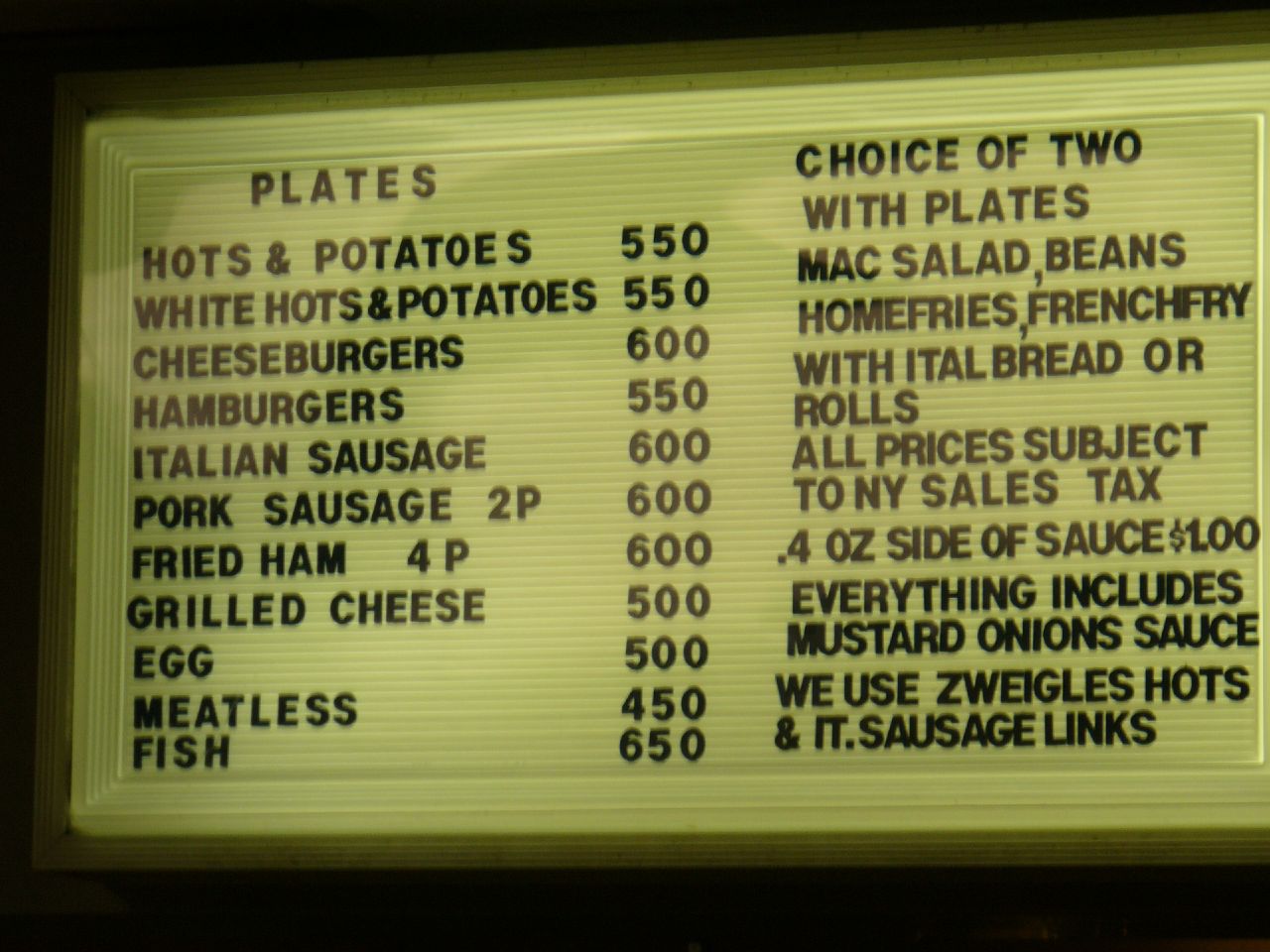**Menu Board Description:**

The restaurant's menu board is divided into two sections and features a slightly yellowed background, suggesting it was originally white. The black bordering frames the menu, giving it a distinct and classic look.

**Left Side - Plates Section:**
This section lists an array of dishes under the heading "Plates":
- Hot Dogs and Potatoes: $5.50
- White Hot Dogs and Potatoes: $5.50
- Cheeseburgers: $6.00
- Hamburgers: $5.50
- Italian Sausage
- Pork Sausage
- Fried Ham (four pieces)
- Grilled Cheese Sandwich
- Egg Plate
- Meatless Dish
- Fish Dish

**Right Side - Choice of Two Section:**
Headed with "Choice of Two," this section offers a variety of sides to accompany the plates:
- Macaroni Salad
- Beans
- Home Fries
- French Fries

Inclusive with Italian bread or four rolls, this side clearly highlights customer choices for a complete meal. Additionally:
- All prices are subject to New York sales tax.
- A four-ounce side of sauce is available for $1.00.

All meals come with mustard and sauce, and the menu proudly states the use of Zweigel's Hots and Italian sausage links.

This thoroughly detailed menu invites diners to enjoy a variety of wholesome, classic dishes in a charming and traditional restaurant setting.